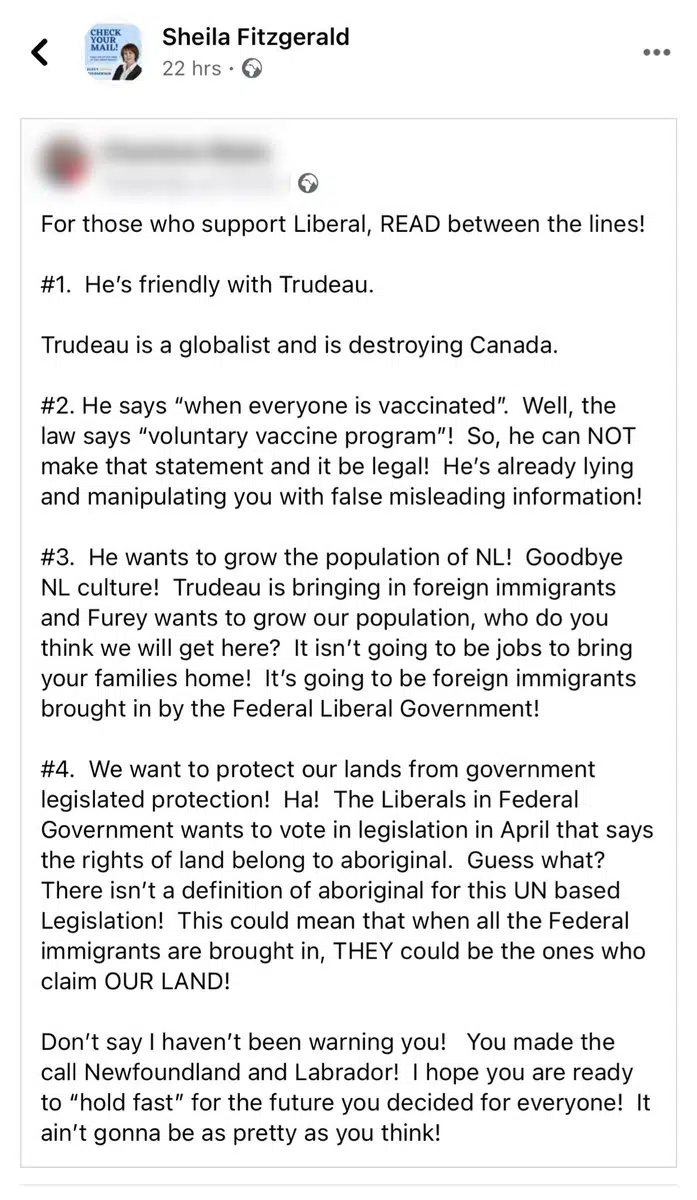Here's a detailed and cleaned-up caption for the described social media post:

---

**Post by Shyla Fitzgerald:**

*Profile Picture:* A small image of a woman in a formal outfit set against a blue background with unreadable text to her left.

*Platform:* Unknown (possibly Facebook)

*Post Details:*
- **Timestamp:** Posted 22 hours ago
- **Visibility:** Publicly shared (indicated by an earth symbol)
- **Navigation:** There's a left-pointing arrow for going back and a three-dot settings menu on the right.

*Reposted Content:* 
- **Original Author:** Blurred out.
- **Text Content:**
  - **Title:** "For those who support Liberal, read between the lines."
  - **Bullet Points:**
    1. "He's friendly with Trudeau. Trudeau is a globalist and is destroying Canada."
    2. "He says, 'when everyone is vaccinated,' while the law states it's a voluntary vaccine program, making this statement legally false. He's already lying and manipulating you with misleading information."
    3. (Not specified)
    4. (Not specified)

*Summary:* Shyla Fitzgerald has reposted a politically charged message criticizing liberal viewpoints and highlighting perceived inconsistencies in statements about vaccination policies connected to Canadian Prime Minister Trudeau.